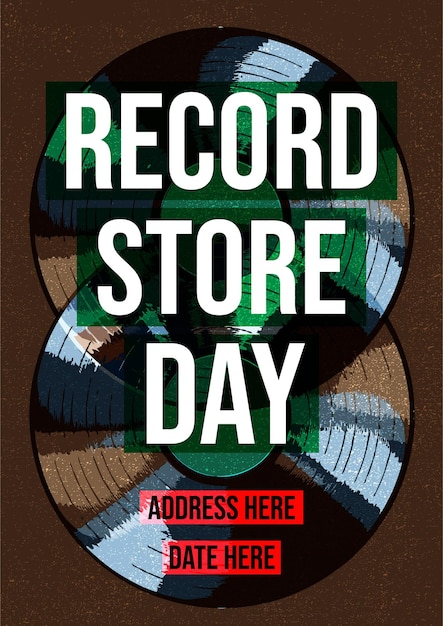This is a detailed description of a poster designed to advertise a Record Store Day event. The poster has a brown background and prominently features two vinyl records in the center that exhibit a camouflage-themed palette with colors such as brown, white, black, gray, dark midnight blue, and lighter blue. The vinyl records are arranged in a way that resembles the number 8. Dominating the center of the poster, large block letters in white spell out "Record Store Day" over three lines. Each line of text is framed by a green background, making the letters stand out. Below this, two lines of text are highlighted with red labels, and these placeholders read "Address Here" and "Date Here" in black writing. The overall aesthetic of the poster is earthy and warm, incorporating many brown and green tones. Designed as a template, this poster allows customization for any record store's event, but in its current form, it contains no specific identifying details.